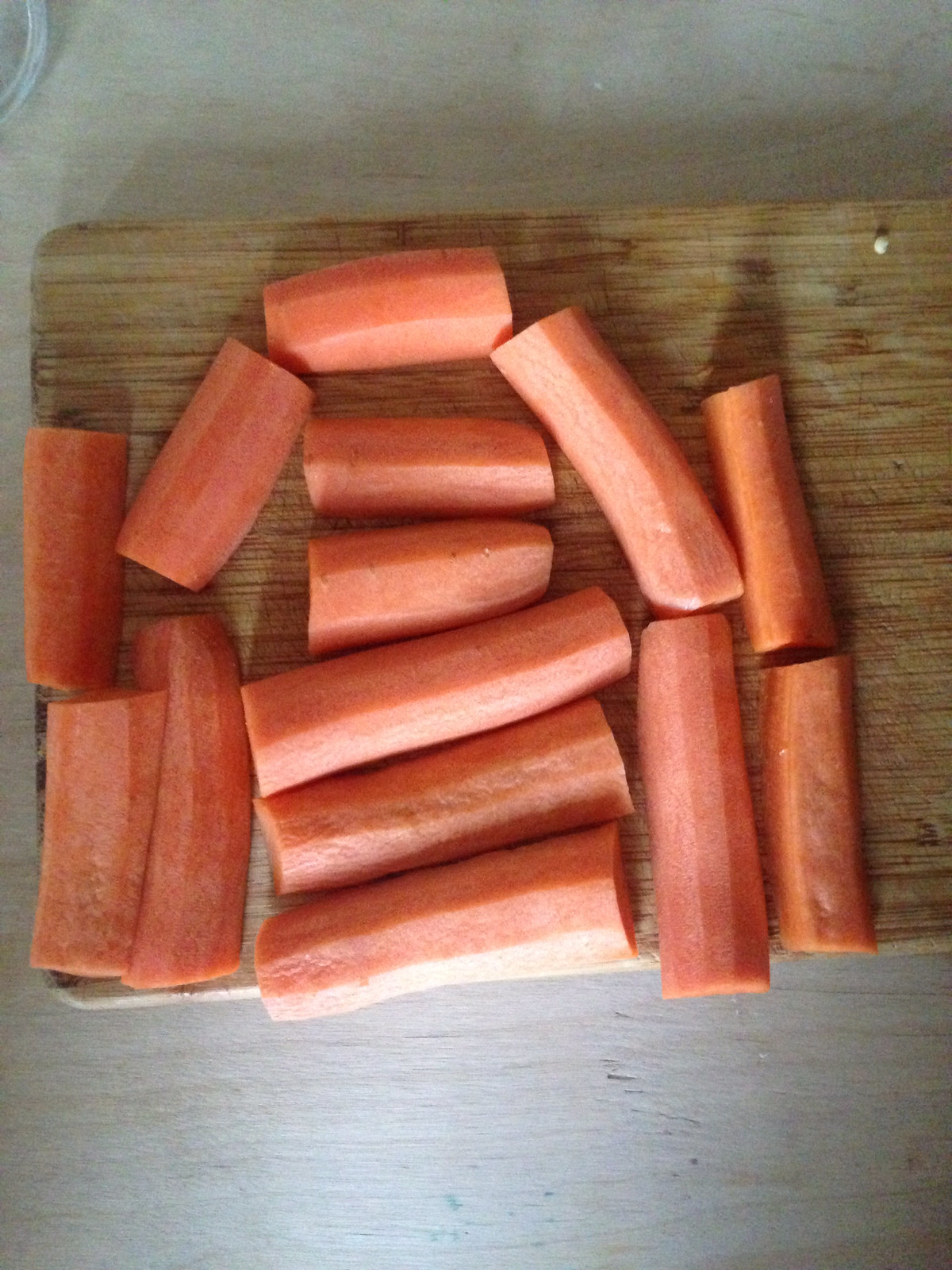The color photograph captures a bird's eye view of a small, dark wooden cutting board sitting on a light gray countertop. Positioned roughly in the middle of the image, the cutting board is scattered with 14 uniformly chopped carrot segments, all of them displaying their solid orange interiors. These medium-to-large carrots have been sliced roughly in half or in thirds, with the ends removed. The arrangement on the cutting board features approximately half of the carrot pieces aligned horizontally and the other half vertically. A small white crumb is noticeable in the top right corner of the board. The scene is presented in a highly detailed, close-up portrait mode, emphasizing the clear textures and colors of the carrots and the wooden board.